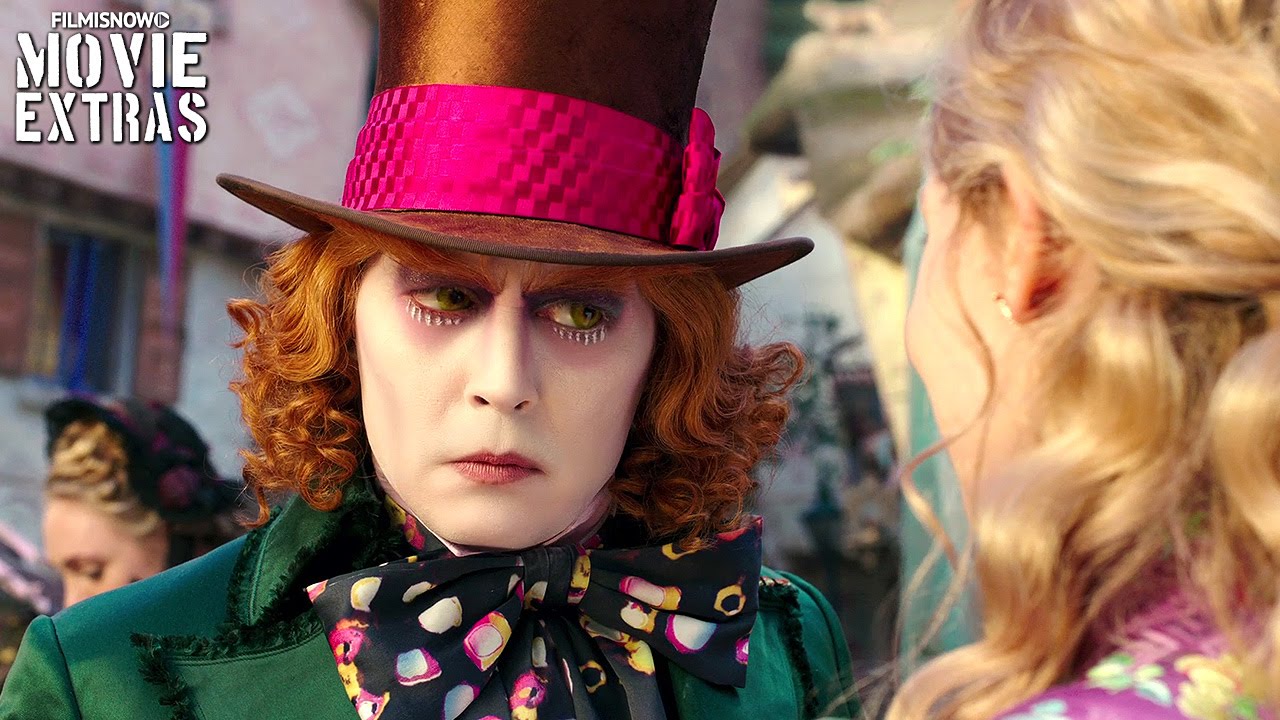This image is a scene from the movie "Willy Wonka," featuring Johnny Depp in the central role. At the very center is Willy Wonka, a man with pale skin, long curly reddish-orange hair, and a black top hat adorned with a pink ribbon. He is heavily made up with white makeup, red eyeshadow, and lipstick. Wonka is dressed in a vibrant green coat paired with a black bow tie adorned with colorful designs, including cats in various hues such as white, pink, and yellow. He stands staring intensely at a woman with blonde hair and a light complexion, who is dressed in a purple blouse or dress and appears to be wearing earrings. In the background, there are several other people walking across a building, suggesting a bustling atmosphere. The scene is well-lit, indicating either daytime or strong artificial lighting. The top left corner of the image features text that says "Movie Extras," emphasizing its connection to film production.